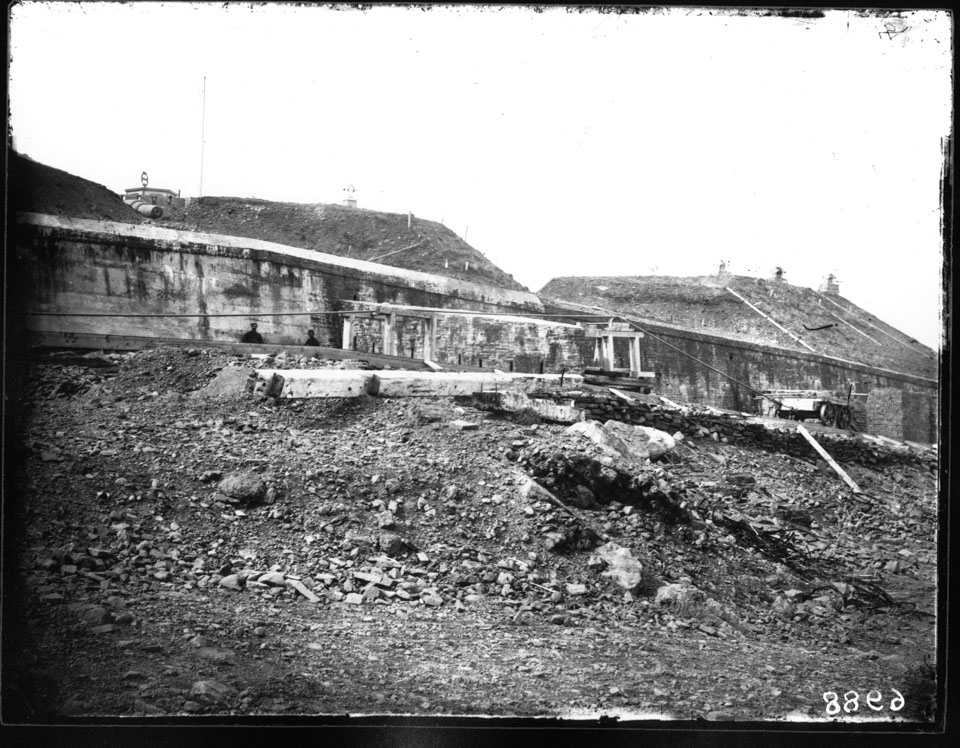This black-and-white photograph captures a scene that appears to be a war-torn or disaster-stricken area located on a mountainside. The foreground is dominated by piles of dirt, rubble, and debris, including pieces of wood and rocks scattered across the landscape. The composition includes a cart with wagon wheels, positioned against a backdrop of a stone wall, beyond which lies a concrete retaining wall. On the retaining wall stand the silhouettes of two men.

The shot depicts mounds of earth above the retaining wall and a road or path running parallel to it. In the background, partially obscured by the chaotic foreground, are two houses and an antenna pole behind the house on the left. The sky above is a stark, bright white, which contrasts sharply with the grayscale landscape below, enhancing the somber and desolate mood of the image. In the bottom right-hand corner, the image is marked with the notation "88ED."